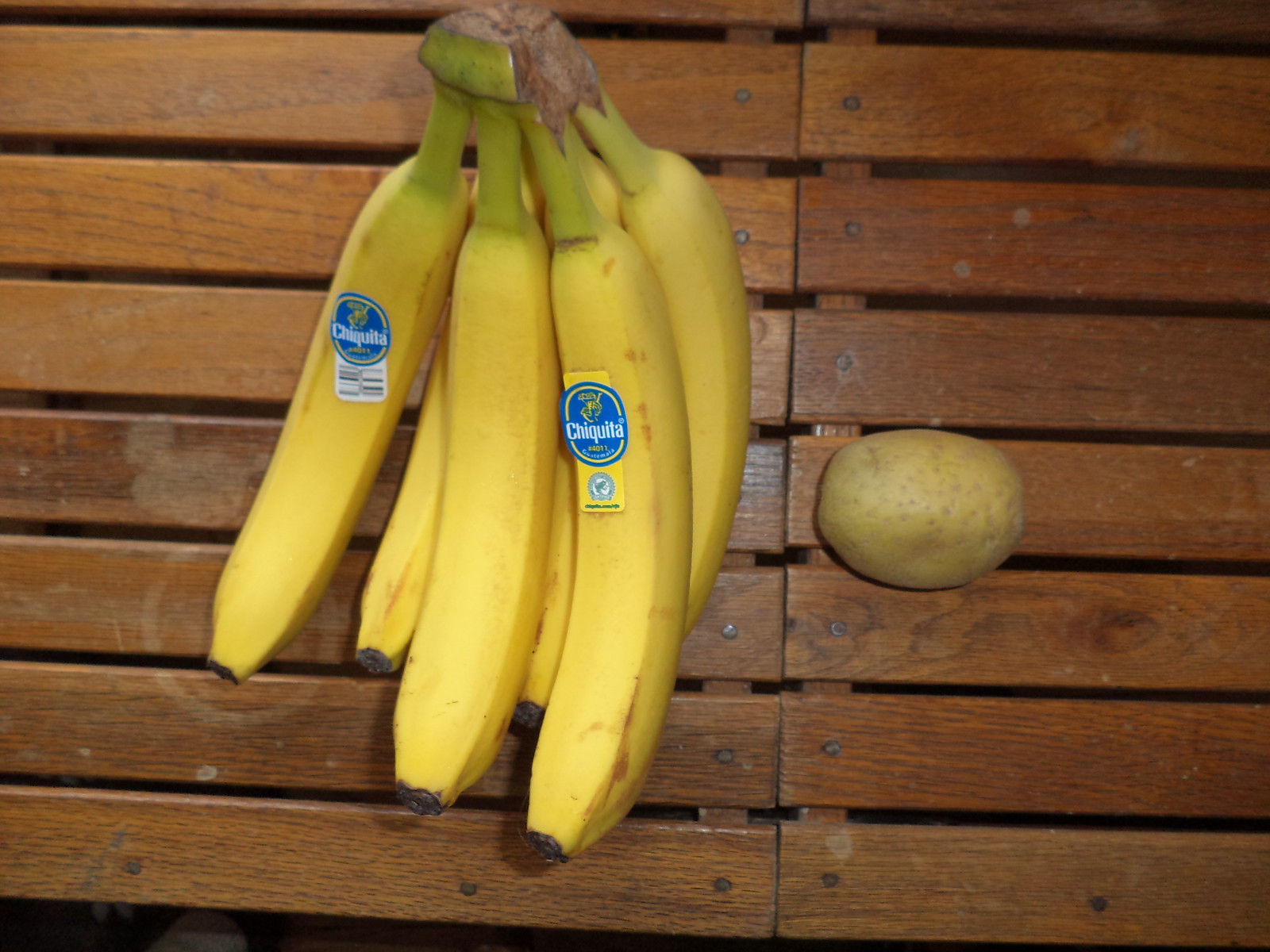A digital photo captures what appears to be an indoor or outdoor setting, featuring a dark, rich brown wooden table composed of wide slats. The background behind the table appears pitch black. The table seems to be made up of two separate tables pushed together, as indicated by a distinct vertical slit slightly right of center, running the entire length of the image. In the lower center, the table ends, creating a black slit that narrows diagonally from left to right, ending at the bottom right corner.

On the left side of the table, there is a bunch of bananas. The top of the bunch is a vibrant green where the bananas grow together, while the cut end is browned out. The bunch includes three bananas in the back that transition from green to yellow, and three in the front. The front-left banana starts green and turns yellow, while the other two are predominantly yellow with green stems. One of these bananas features a Chiquita sticker, a blue oval with a yellow woman in a banana hat and the word "Chiquita" in white, along with a black barcode. Another banana has a similar Chiquita sticker with an additional orange rectangle attached, containing some white text at the bottom.

On the far left, the wood shows a white ring stain, likely from a coffee cup or mug. Closer to the center-right on the adjacent table, there is a tan-colored, oval-shaped potato.